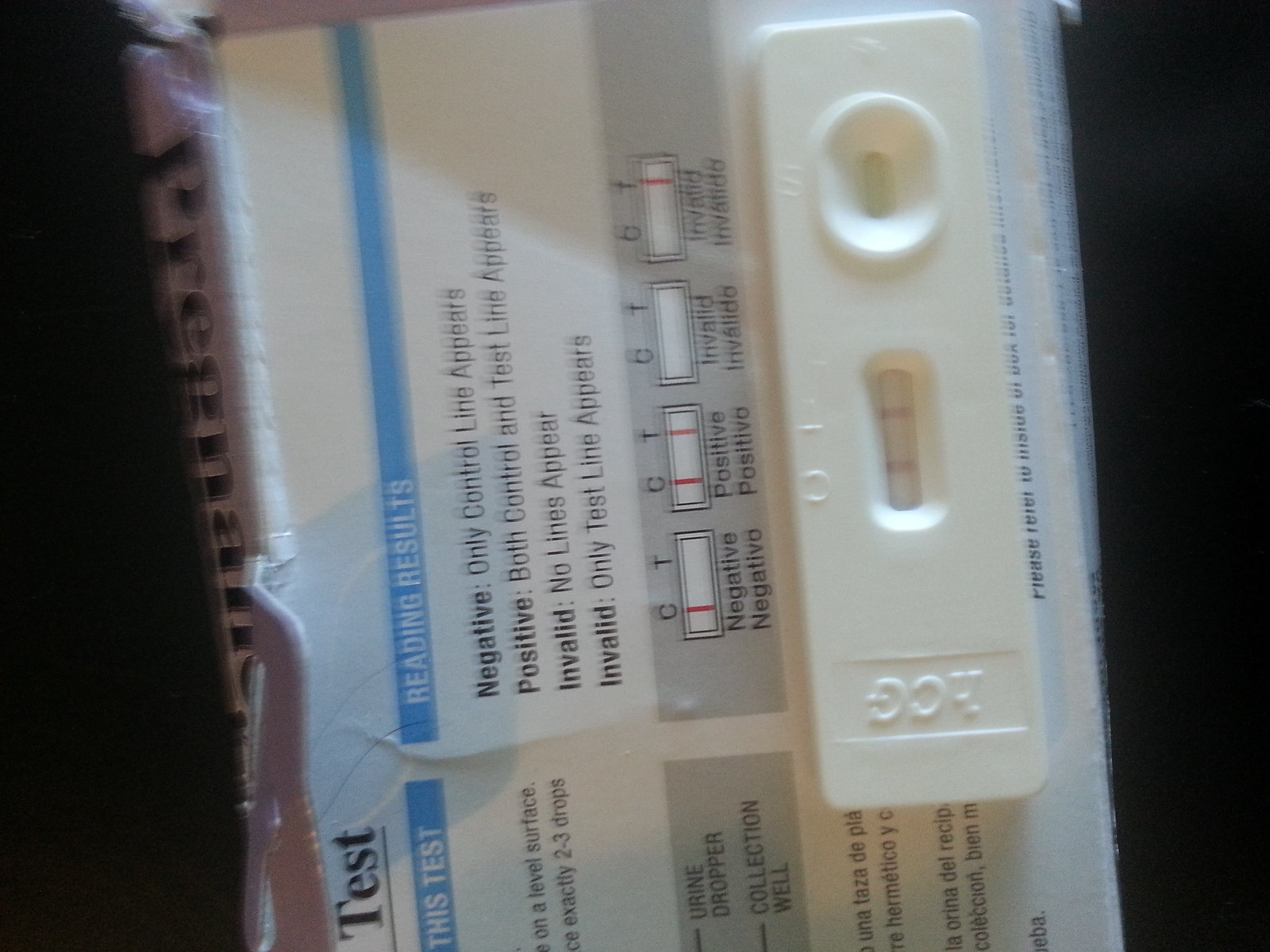The image depicts a slightly damaged pregnancy test package against a black background. The left side of the package shows the word "pregnant," confirming it is indeed a pregnancy test. The package is a bit beat up and has been partially torn open, revealing its contents. On top of the white box lies a white pregnancy test stick labeled with "HCG" at the bottom. The test features a small window indicating the results, currently displaying two pink stripes, signifying a positive result.

The front of the box is white with a bright blue strip containing white text that explains how to read the test results. It states:
- Negative: Only the control line (C) appears.
- Positive: Both the control (C) and test (T) lines appear.
- Invalid: No lines appear.
- Invalid: Only the test line (T) appears.

Illustrations next to the text show examples of each result type:
- Negative: One red line on C.
- Positive: Red lines on both C and T (matching the visible result in the test window).
- Invalid: No lines or only a line on T.

Additional text on the box explains instructions like "level surface," "exactly two drops," "urine dropper," and "collection well." Instructions in Spanish are also visible on the package.